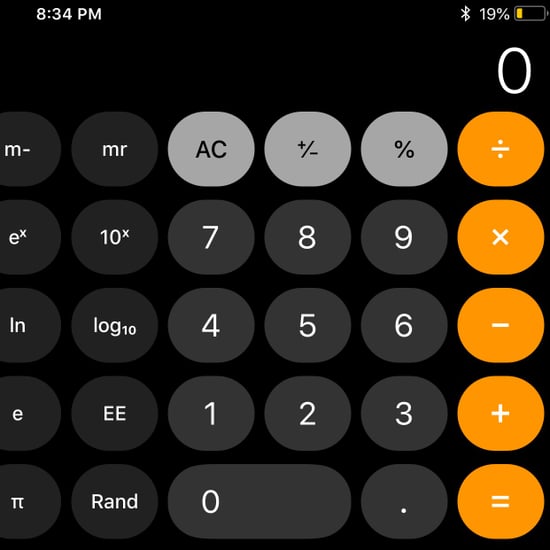The image displays a smartphone screen showcasing a calculator app with a dark theme. At the top left corner, the time is displayed as 8:43 PM, while the top right corner shows the Bluetooth icon and a battery level indicator at 19%. The calculator itself features a dark black background. The numeric buttons and symbols are in varying shades of gray, with lighter gray used for some and darker gray for others. The primary mathematical operation symbols—division, multiplication, subtraction, addition, and equals—stand out in bright orange. Currently, the calculator is idle, showing just the number zero in white. Additionally, the interface includes advanced functions like M-, MR, exponent, and 10 log, all in darker gray, indicating the availability of more sophisticated features rather than just basic calculations.